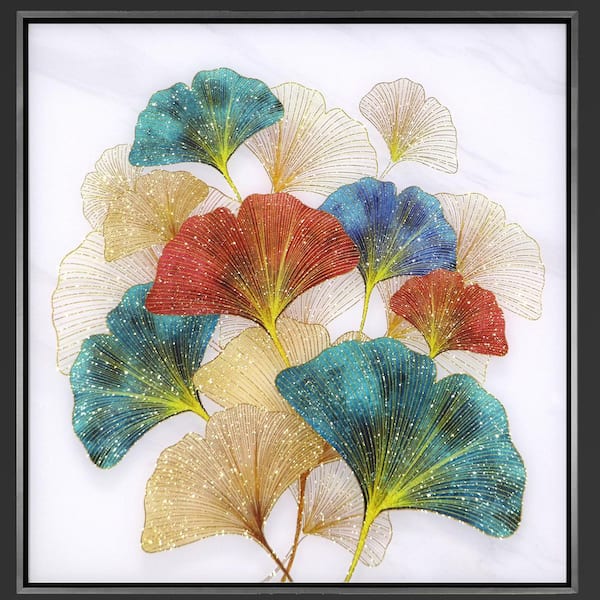The image features a sophisticated and vibrant painting encased in a dark grey photo frame with a deeper black outline as a border. The painting has a predominantly white background with hints of light blue, reminiscent of wispy clouds. Central to the artwork are 10 to 15 semi-circular, leaf-like shapes in an array of colors, including blue, dark blue, light green, red, white, and cream. Each leaf displays vertical yellow lines that connect to an elongated yellow base, giving them a dynamic appearance. The leaves appear almost to shimmer, as if embossed with glitter or a powdery, starlight-like texture, adding to the overall fanciness and luminous quality of the piece.